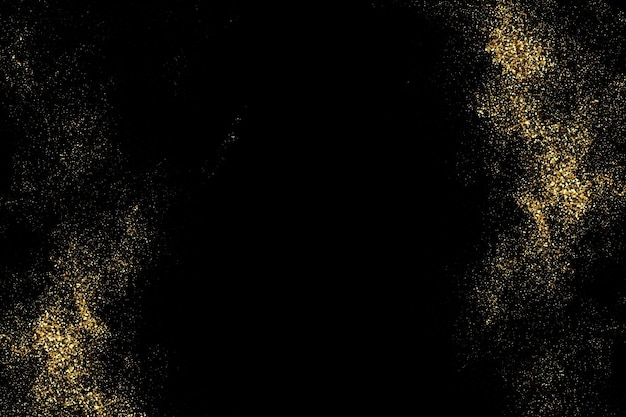The image is a rectangular piece, wider than it is tall, featuring a primarily black background. The darkest area is in the center, creating an almost pitch-black void. Along the sides, numerous golden speckles are scattered, giving the appearance of celestial stars. These specks are most concentrated in the bottom left corner, top right corner, and middle right side, creating a beautiful, contrasting effect of gold against black. The pattern of speckles diminishes towards the center, further enhancing the image's stark, cosmic feel. While it doesn't resemble anything specific, the image exudes a sense of night-time sky or a starry night, possibly even suggesting a computer-generated graphic or abstract painting.